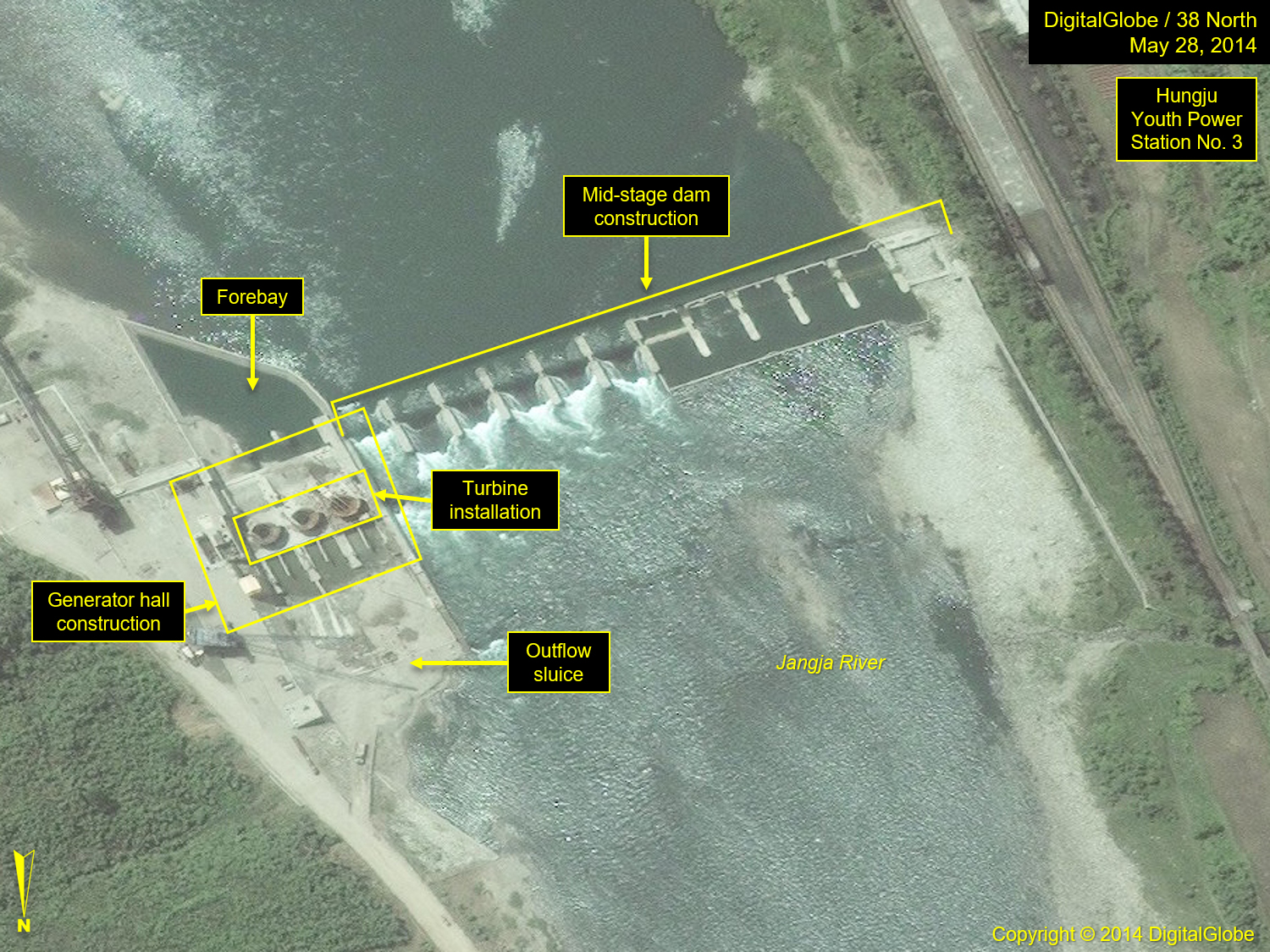The aerial image, a satellite photograph labeled "Digital Globe / 38 North May 28, 2014," provides a detailed view of the Hunjoo (Hangzhou) Youth Power Station Number 3. The photo shows the ongoing mid-stage construction of a large dam spanning the Janja River, which runs centrally through the image. Forested areas dominate the lower-left section, while the right side is sparsely vegetated closer to a visible road. Key structures are annotated with yellow text and arrows, such as the forebay, generator hall construction, turbine installation marked by three donut-shaped structures, and the outflow sluice channeling water from the dam. The alluvial soil along the river's edge suggests a floodplain area. The directional compass indicates that north is at the bottom of the image. Copyright information, "2014 Digital Globe," is noted in the bottom right corner.